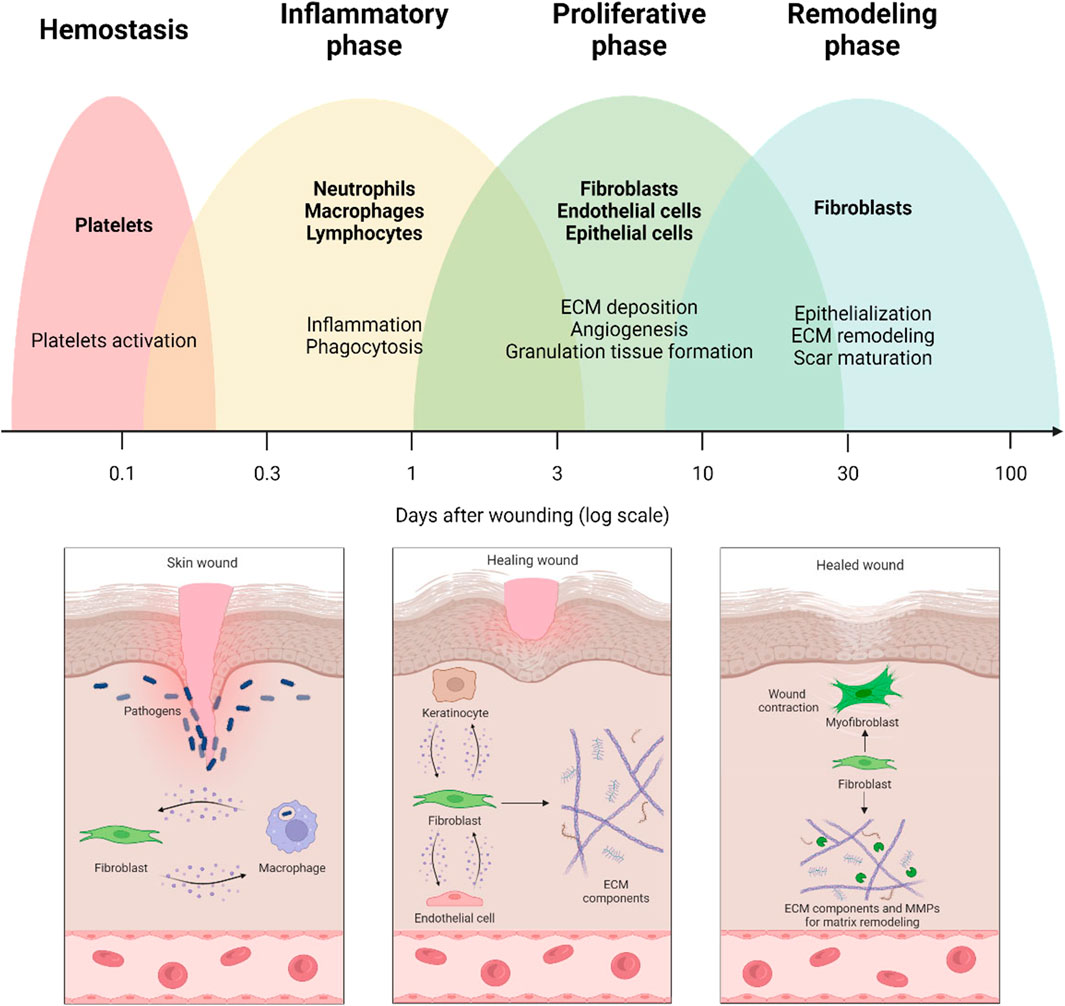The image is a detailed medical chart commonly found in textbooks, illustrating the different phases of wound healing. The chart is divided into a top and bottom half. The top half features a horizontal timeline marked from 0.1 to 100 days post-wounding, with phases labeled: Hemostasis, Inflammatory Phase, Proliferative Phase, and Remodeling Phase. Each phase is represented by overlapping half-circle shapes in pink, yellow, green, and blue respectively, and contains key information in black text. The Hemostasis phase notes "platelets and platelet activation", the Inflammatory phase includes "neutrophils, macrophages, lymphocytes, and inflammation phagocytosis", the Proliferative phase mentions "fibroblasts, endothelial cells, epithelial cells, ECM deposition, angiogenesis, and granulation tissue formation", and the Remodeling phase highlights "fibroblasts, epithelialization, ECM remodeling, and scar maturation".

The bottom half of the image contains three rectangular panels displaying side views of skin at various healing stages. The first panel, labeled "skin wound", shows a fresh wound with pathogens and includes a visual of fibroblasts and macrophages within a pink layer. The second panel, labeled "healing wound", depicts the wound partially closed with active keratinocytes, fibroblasts, endothelial cells, and ECM components aiding in the healing process. The final panel, labeled "healed wound", illustrates a fully healed skin surface with references to wound contraction involving myofibroblasts, fibroblasts, ECM components, and MMPs for matrix remodeling. The entire image is set against a plain white background, typical of educational medical posters.